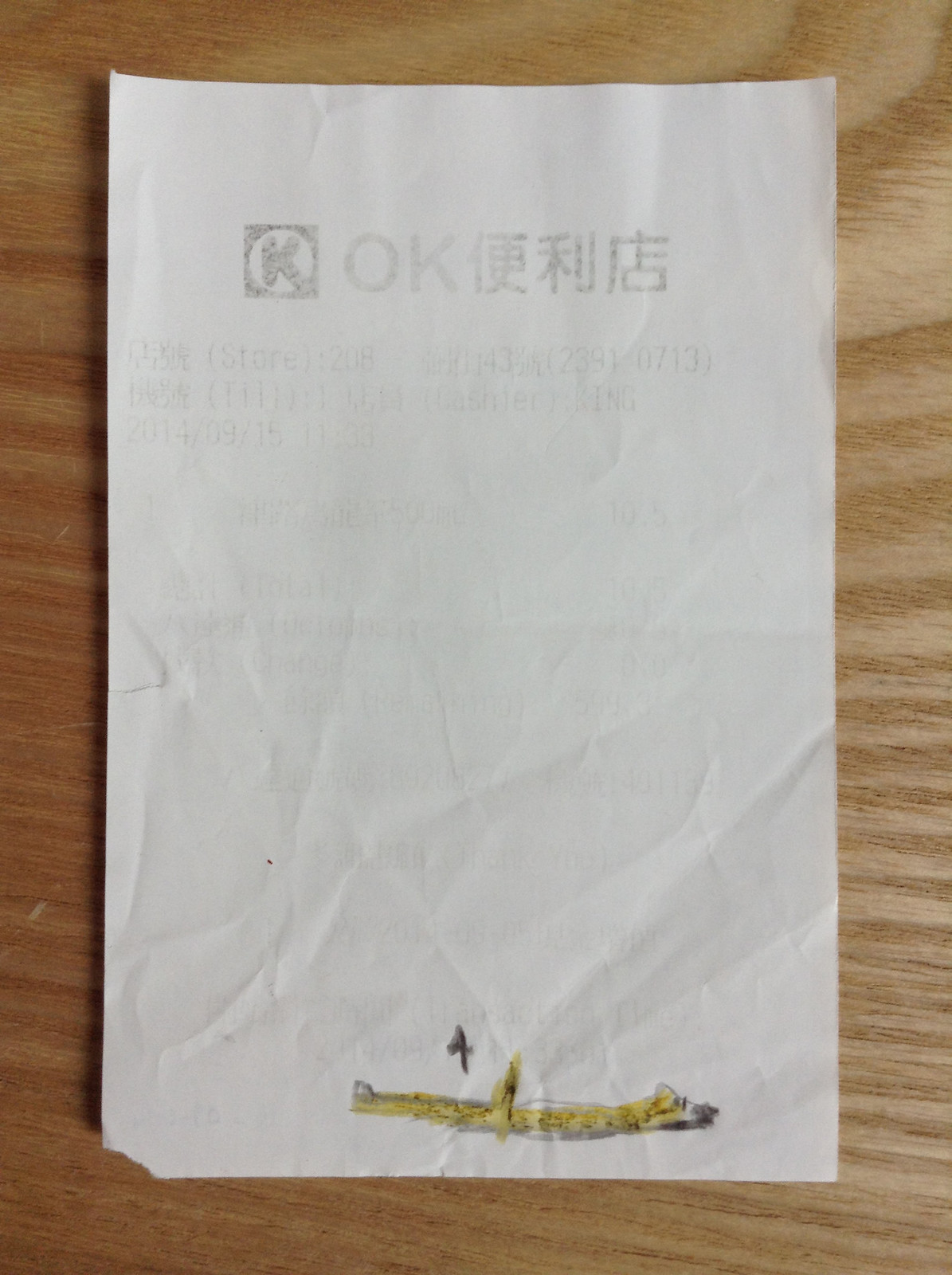A short, faded receipt sits on a desk with a tan-colored, ingrained wood background. The text at the top of the receipt is mostly worn away, but the letters 'K' and 'OK' are still visible, followed by three Japanese characters. The rest of the writing is too faint to decipher. The bottom portion of the receipt features a noticeable stain or rip that spans roughly half its width, adding to its worn appearance.